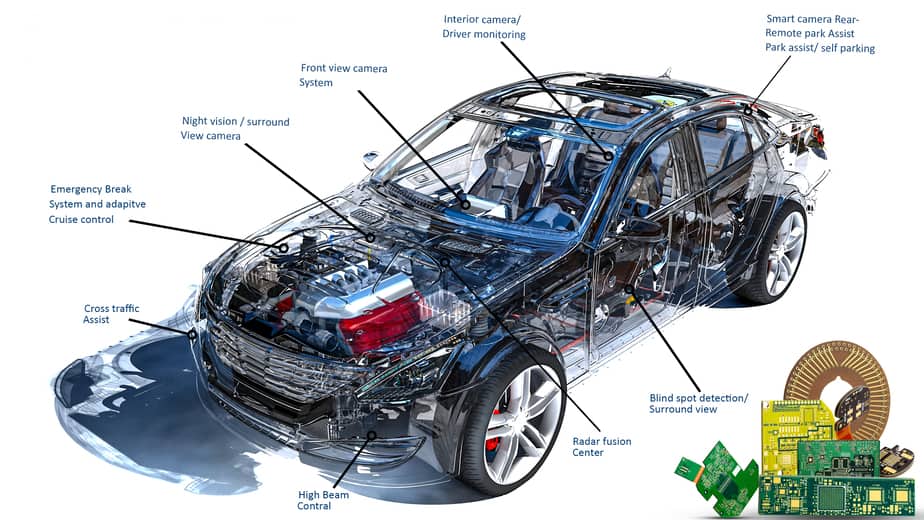The image showcases a detailed diagram of a mostly transparent car, allowing a clear view of its interior components, including the engine and seats. Various parts of the car are meticulously labeled with blue text and black guiding arrows. Key features identified include high beam control, cross traffic assist, emergency brake system, adaptive cruise control, night vision surround view camera, front view camera system, blind spot detection, radar fusion center, interior camera, driver monitoring, smart camera rear remote, park assist, and self-parking capabilities. Additionally, in the bottom right corner, there are illustrations of electronic circuits and microchips. The car itself is predominantly depicted in blue and black, set against a white background.